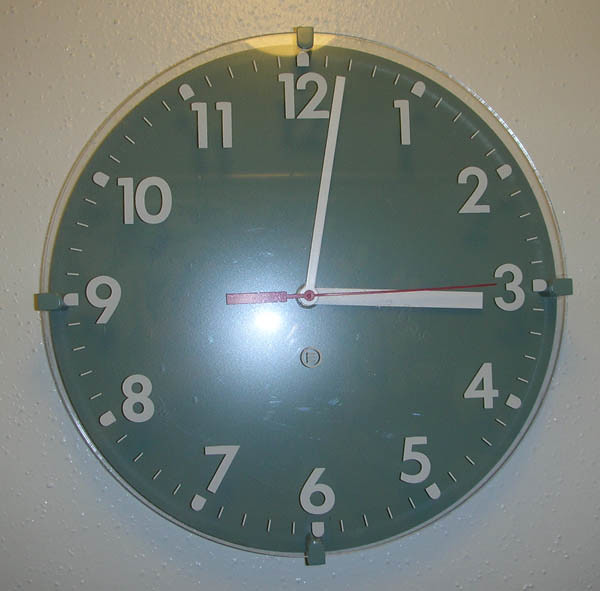This image captures a standard wall clock set against a vibrant green background. The clock features bold white numerals and hands that stand out clearly, indicating the time as 3:02 PM. The clock face is transparent, allowing a faint reflection of a lamp to be seen through the glass cover. At the center of the clock, a small golden 'F' adds a unique touch to its otherwise minimalist design. Its simple and inexpensive appearance suggests it is a commonly found clock, widely available in many retail stores.